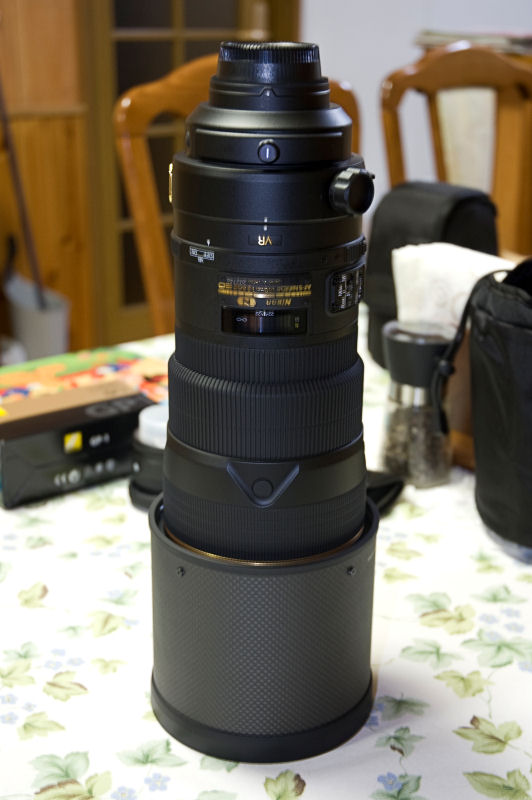This photograph features a detailed up-close shot of a detached, long Nikon DSLR camera lens lying vertically on a table with a floral-themed tablecloth. The lens, which is fully extended and approximately a foot long, has a matte black body with a gray base around the glass element. There are several toggles and buttons for adjusting settings and a ridged focus ring for a better grip. A protective plastic cover can be seen near the eyepiece where the lens attaches to the camera. The background includes a pair of polished brown wooden chairs and a wooden cabinet with a glass-fronted door, adding a homey, lived-in feel to the scene. Additionally, a black camera bag is visible to the right of the lens, while an ambiguous box sits to the left. The setup resembles a product listing photo, suggestive of an item being shown for sale.